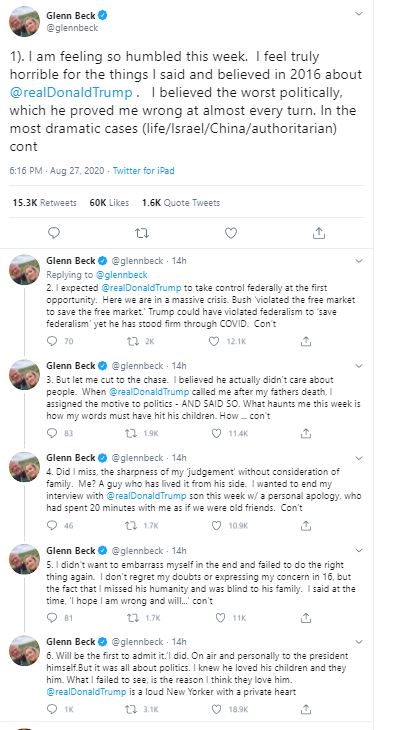This is a screenshot of a tweet from the Twitter page of Glenn Beck. In the upper left-hand corner, there is his profile picture with his name, "Glenn Beck," above his handle, "@glennbeck." The tweet reads: 

"I am feeling so humbled this week. I feel truly horrible for the things I said and believed in 2016 about @realDonaldTrump. I believed the worst politically, which he proved me wrong at almost every turn, in the most dramatic cases like Israel, China, and authoritarianism."

The tweet was written and published on August 27, 2020, at 6:16 p.m. Below the tweet, there is a series of five replies that Glenn Beck wrote in response to various comments on his post.